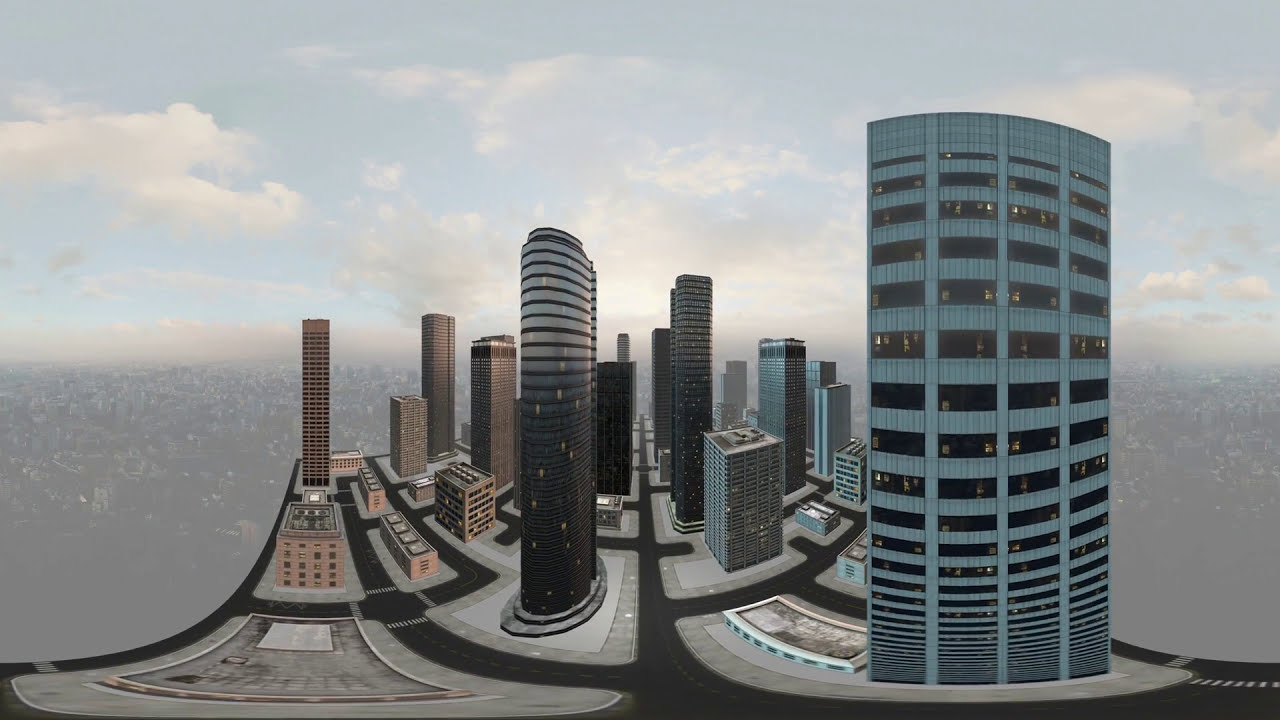This computerized artwork depicts a digitally rendered cityscape, featuring a complex network of roadways leading into a cluster of both tall and shorter buildings. Dominating the center of the image are skyscrapers, ranging between 20 to 30 stories high, that showcase illuminated windows. The scene appears to be viewed from an elevated perspective, possibly a mountaintop, giving the impression of a city built atop another sprawling urban landscape. The sky is a very pale blue adorned with white clouds, indicating a daytime setting without visible sunshine. The color palette includes shades of blue, black, gray, white, and brown. Despite the intricate roads and interconnecting pathways around and within the city, there are no cars or textual markers identifying the location or artist, enhancing its resemblance to a scene from a video game.